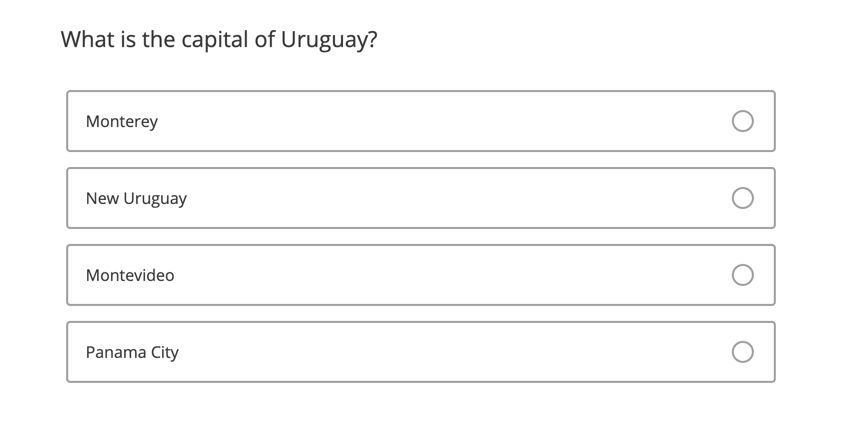The image depicts a question from an online test or quiz, featuring a dark gray background at the top left corner with the question presented in the same color font: "What is the capital of Uruguay?" Below the question, there are four long rectangular boxes containing the answer choices, also written in dark gray font. The options listed from top to bottom are:

1. Monterey
2. New Uruguay
3. Montevideo
4. Panama City

To the right of each answer choice is a small circular button, presumably for selection purposes. The layout is clean and straightforward, designed for easy readability and interaction.